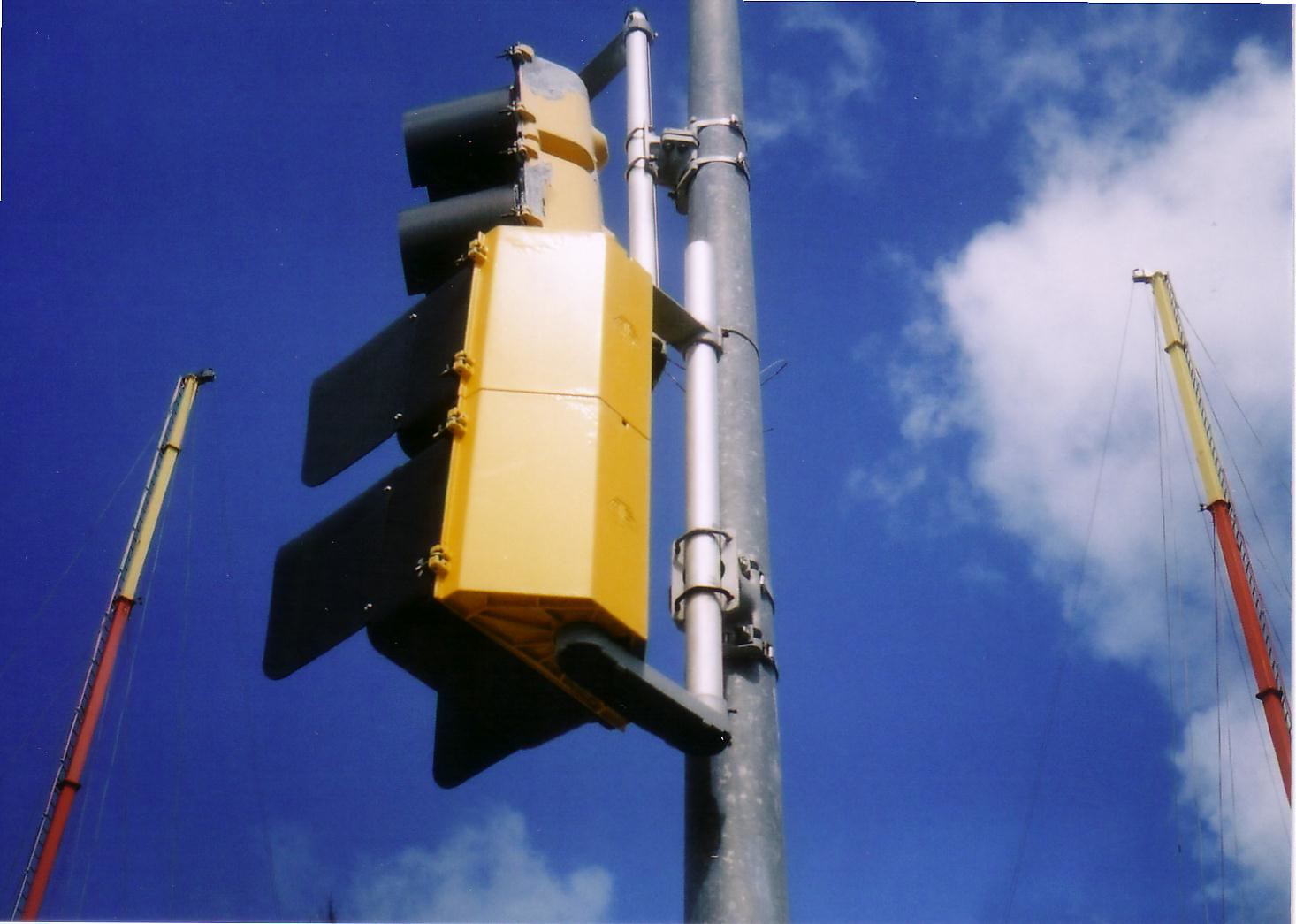This square photograph captures an upward view of the back of a yellow stoplight, meticulously detailed and defined against a vibrant blue sky embellished with fluffy white clouds. The stoplight itself showcases four lights on its front side and features rounded black covers on the top and flat black covers at the bottom. It is suspended from a complex assembly of poles and brackets; a silver pole is perched horizontally above the stoplight, secured with a bracket near the stoplight's top. Additionally, a vertical pole to the left mounts the stoplight with sturdy brackets at both the top and bottom, the latter appearing as a thick, grey plastic pole. These smaller poles and brackets are further reinforced by a larger, overarching silver pole. 

The setting surrounding the stoplight adds to the intricacy of the scene, with ship masts visible on both the left and right sides, hinting at a nautical environment. Red and yellow metal poles are interspersed within the composition, contributing to a dynamic and industrial aesthetic. The vivid details of the stoplight's structure and its various supporting elements are accentuated by the crisp, clear sky, which provides a picturesque and serene backdrop to this urban mechanical ensemble.